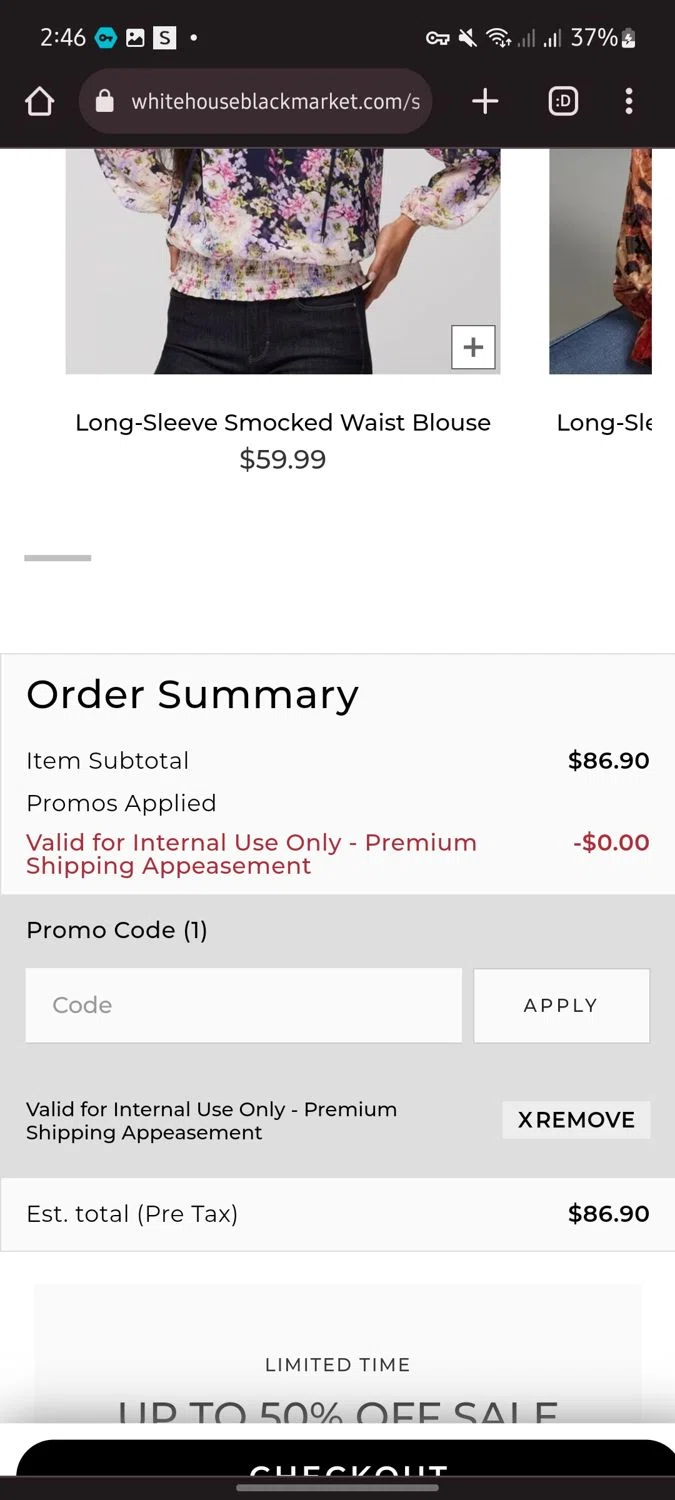This image is a detailed snapshot of the checkout page on the website whitehouseblackmarket.com. At the top of the page, the browser's address bar prominently displays the website's URL. The central focus of the webpage showcases an image of a woman wearing a floral-patterned blouse priced at $59.99. Directly below the image, an order summary is presented, detailing a subtotal of $86.90 with the option to enter a promo code, which currently remains blank. The summary also includes the estimated pre-tax total, consistent at $86.90. Occupying the lower section of the page is a prominent black checkout button with 'Checkout' written in white font. Above this button, a banner announces a limited-time sale, offering discounts up to 50% off. The website design features a minimalist aesthetic with a white background and predominantly black text. Additionally, the cell phone's battery indicator in the top-right corner reads 37%.